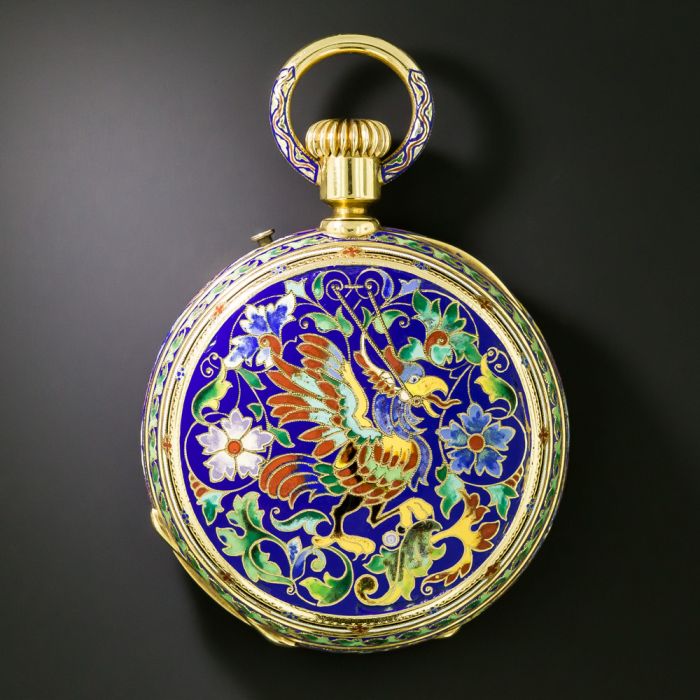This captivating image features a gold pocket watch, vividly adorned and set against a subtly shaded black backdrop, which lightens to a gray hue on the left. The pocket watch, with its circular body and a top knob, showcases an intricately colorful design reminiscent of a stained glass window. The central motif is a striking, semi-cartoonish peacock in mid-strut, its right foot on the ground and its left foot raised. The bird's feathers are an elaborate blend of red, yellow, light green, dark green, and blue, with the tallest tail feathers arching proudly above its head. The peacock’s head is blue with expressive eyes, a yellow beak partially open to reveal a curving red tongue, and a pronounced red ear. Surrounding the peacock are swirling patterns of deep blue, green, and yellow, interspersed with white and blue flowers with red centers. The design extends to the watch’s rim, which features similar elaborate patterns. The pocket watch includes a small button on the upper left which, along with a larger ridged knob on top, adds functional detail. This knob, golden and textured, is encased within a ring that also features multicolored accents. The detailed craftsmanship and radiant colors make this pocket watch a mesmerizing piece of art.